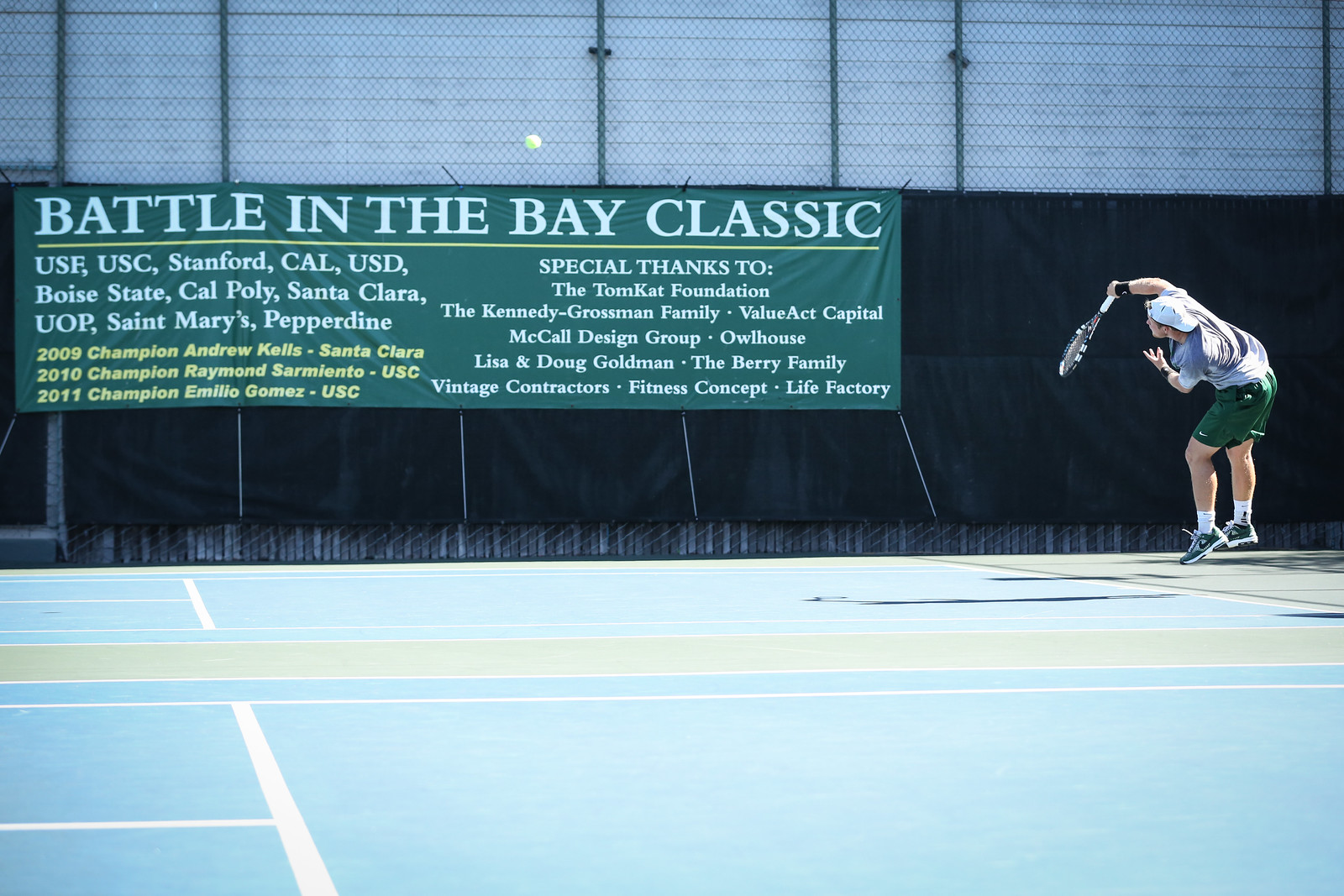This detailed caption combines all the inputs into a cohesive and vivid description:

"A photograph captures a young Caucasian man in the midst of playing tennis on a bright, late evening. He is preparing to return a ball that is mid-air, positioned slightly to the left of center in the image. The player is dressed in a grey shirt, dark green shorts, white tennis shoes, and a white cap worn backwards. The tennis court features a blue surface with white lines, bordered by green on the outer edges. Behind the player, a large banner on a black fence prominently displays the names 'Battle in the Bay Classic' and the universities USF, USC, Stanford, Cal, USD, Boise State, Cal Poly, Santa Clara, UOP, St. Mary's, and Pepperdine. The banner further notes past champions: Andrew Kells (Santa Clara, 2009), Raymond (USC, 2010), and Emilio Gomez (USC, 2011). Special thanks are given to the TomKat Foundation, the Kennedy Grossman Family, ValueAct Capital, Macau Design Group, Owl House, Lisa and Doug Goldman, the Berry Family, Vintage Contractors, Fitness Concepts, and Life Factory. The scene is clearly illuminated by daylight, casting long shadows that enhance the dynamic moment of action on the court."